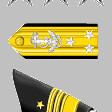The image is a very small photo with a solid gray background. At the center, there's a yellow ribbon adorned with a white embroidered anchor that is oriented sideways, with the bottom of the anchor pointing to the right and the top pointing to the left. Surrounding the ribbon are thin horizontal black stripes on both the top and bottom edges. Additionally, three white stars are arranged beneath the anchor in a triangular pattern. The ribbon has a flat edge on the right side and an arrow-like shape on the left side. Below this yellow ribbon, partially obscured, is a black flag featuring yellow stripes and a yellow star. The precise origin or purpose of the black flag is not clearly identifiable from the image. Overall, the photo captures just three main elements: the gray background, the detailed yellow ribbon with the white anchor and stars, and the black flag with the yellow design.